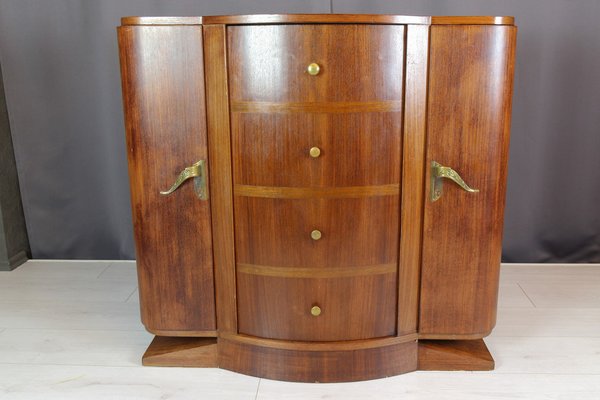In the center of a white-tiled floor with a gray curtain backdrop stands a dark wooden cabinet. This cabinet features four vertically aligned drawers in the middle, each adorned with circular brass handles, summing up to four handles. On either side of the drawers are tall, thin doors that swing outward—one to the right and the other to the left—each equipped with a slightly ornate, curved brass handle. The cabinet sits atop a slightly raised wooden base that seamlessly integrates with its structure. The wood has a slightly reflective quality, capturing light towards the top. The functionality of the top surface remains uncertain, reminiscent of a potential record cabinet.